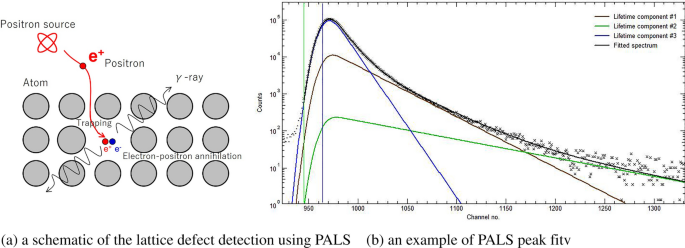The image is a detailed scientific diagram with a predominantly white background. On the left side, there is an illustration featuring grey circles with various annotations. Central to this section is a positron source depicted as two overlapping red 'O's in a star pattern, from which a squiggly line with an arrowhead moves towards the center of the grey circles labeled "atom." There are several terms illustrated within this area, including "trapping" on the red line, "electron-positron annihilation," and a wavy line labeled with a symbol resembling R-ray. The grey circles also contain red and blue dots marked "E+" representing positrons, with one red dot on the moving arrow labeled "E+ positron."

On the right side of the image is a graph, with multiple colored lines that arc upwards and then slope downwards, accompanied by fuzzy dots that start condensed on the left and disperse towards the right. Although the text and numbers on the graph are too small to read, they serve to display data correlations related to the positron source. Underneath, the text reads "(A) Schematic of the lattice defect detection using PALS" and "(B) An example of PALS peak FITV," with PALS in capital letters. This diagram appears to explain the interaction and detection of positrons within atoms, likely intended for educational or scientific research purposes.